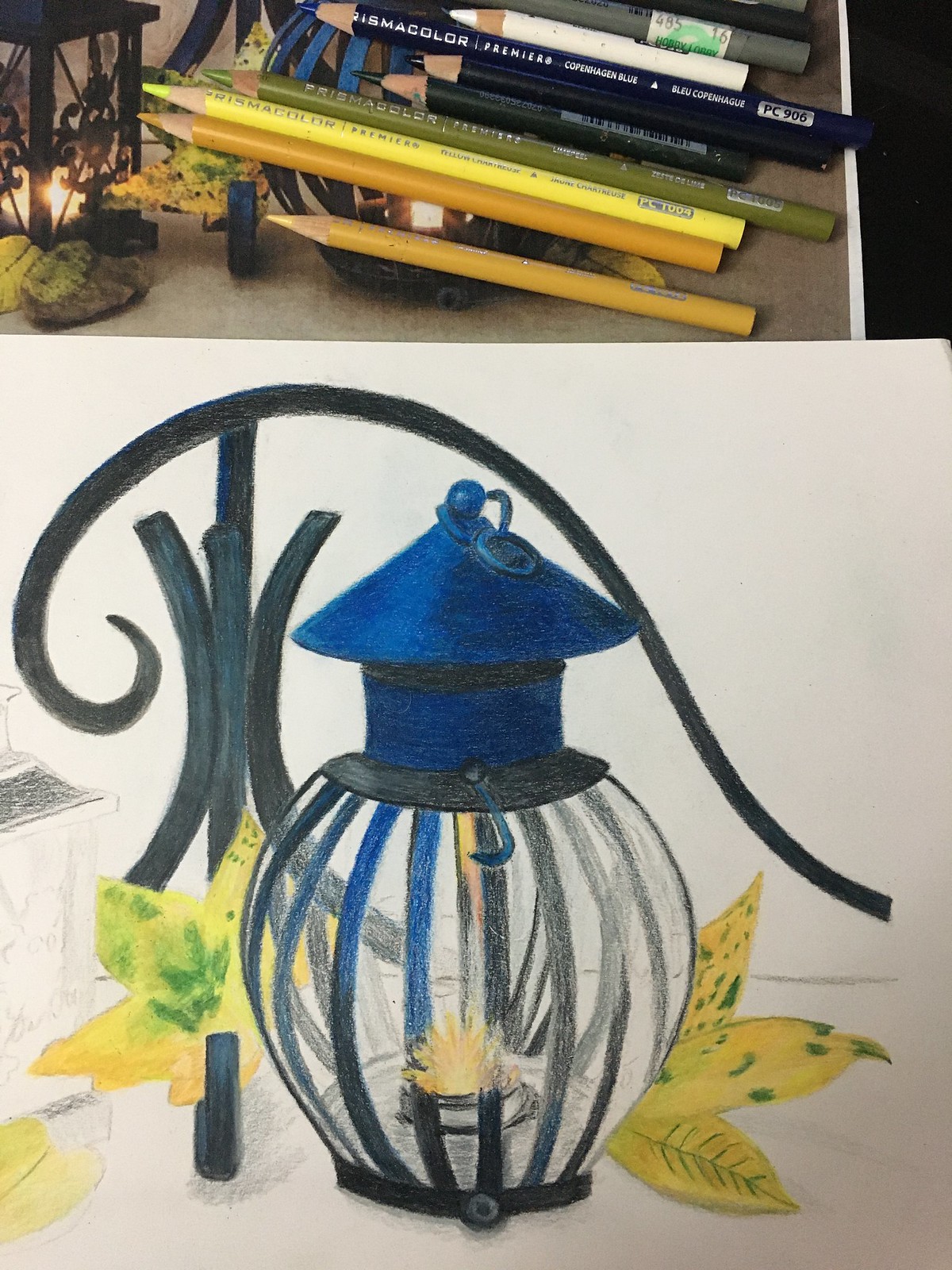A captivating piece of artwork predominantly fills the lower three-quarters of this vertical image, showcasing a lantern illuminated by a warm, flickering light, possibly from a candle or flame. The lantern, illustrated with shades of blue and black, stands against the backdrop of an iron gate, accentuated with scattered leaves on the ground. Above this intricate drawing, an array of colored pencils is meticulously arranged, featuring hues of yellow, gold, green, blue, and white. These pencils likely represent the tools used by the artist to create the vivid and detailed scene below.